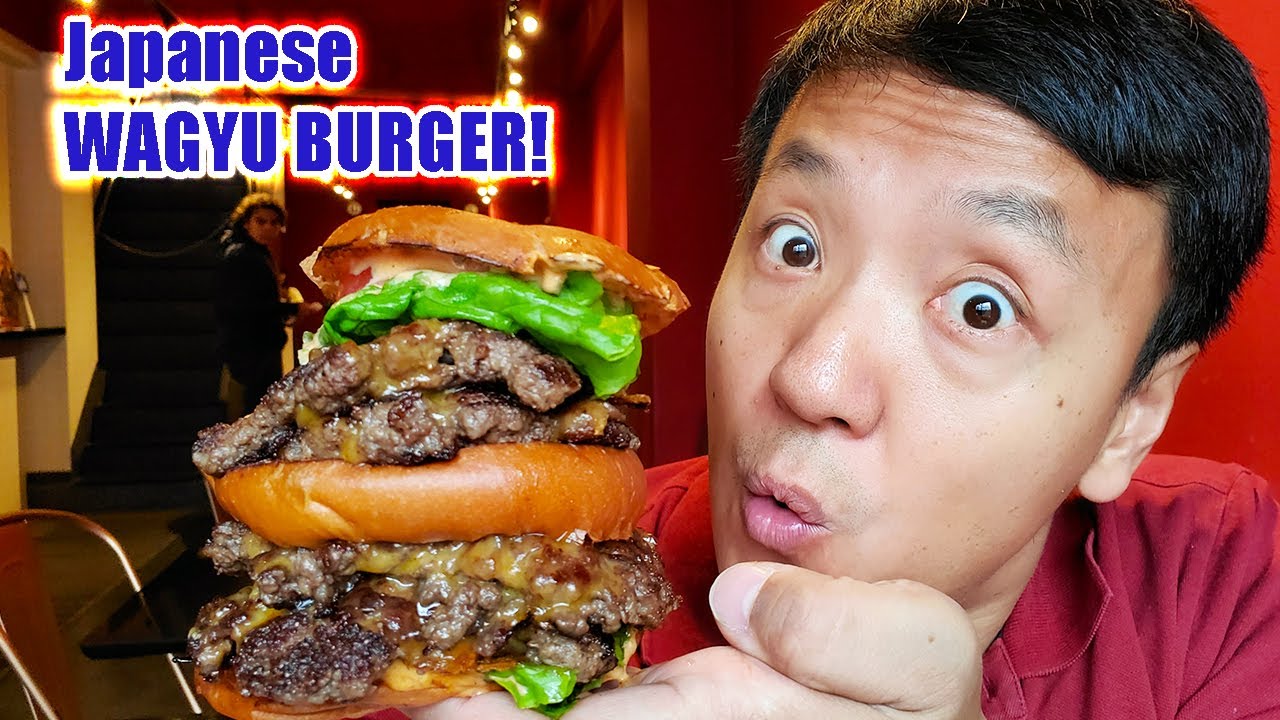In this vibrant and eye-catching image, a social media influencer is seen enthusiastically showcasing a Japanese Wagyu burger. The close-up shot captures the influencer, an Asian man with a surprised expression and wide-open eyes, holding the massive, triple-decker burger in his left hand. The burger is a towering creation, featuring three buns, multiple layers of succulent Wagyu beef patties, melted cheddar cheese, crisp lettuce, and savory bacon. The intricate details of the burger highlight its juicy and mouth-watering appeal.

The background reveals an indoor setting with a dominant red color scheme, enhancing the dynamic and exciting atmosphere of the scene. To the left, a woman is seen walking out the door, adding a sense of movement, while to the right, parts of the restaurant's seating area, including a metal chair, are visible. The text "Japanese Wagyu Burger" is prominently displayed in blue in the upper left-hand corner, making it clear this is an advertisement for the delectable and extravagant burger. The influencer's medium red shirt blends seamlessly with the bright red wall behind him, creating a cohesive and visually striking image that is sure to captivate viewers.